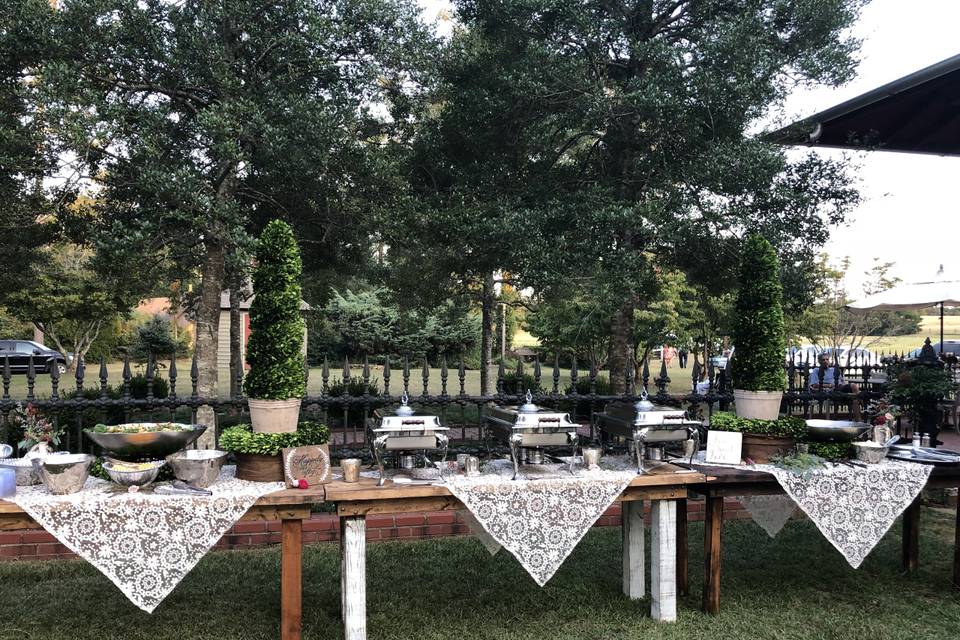This detailed daytime outdoor photograph captures a private event set on an estate, framed by lush greenery and huge trees. In the center of the scene stands a long brown wooden table draped with a lace-type white tablecloth. The table, equipped with white legs in the middle section, features an extensive buffet arrangement with three large chafing dishes heated by Sterno burners, flanked by various bowls, pots, and utensils. Adding to the table's decorative appeal are two conical-shaped plants. The setup is enclosed by a black iron fence and a low brick wall, suggesting a refined, garden-like atmosphere. In the background, beyond the ornate iron gate, a lone black car is parked on a paved area, adding a subtle hint of modernity to this otherwise timeless, serene outdoor celebration.